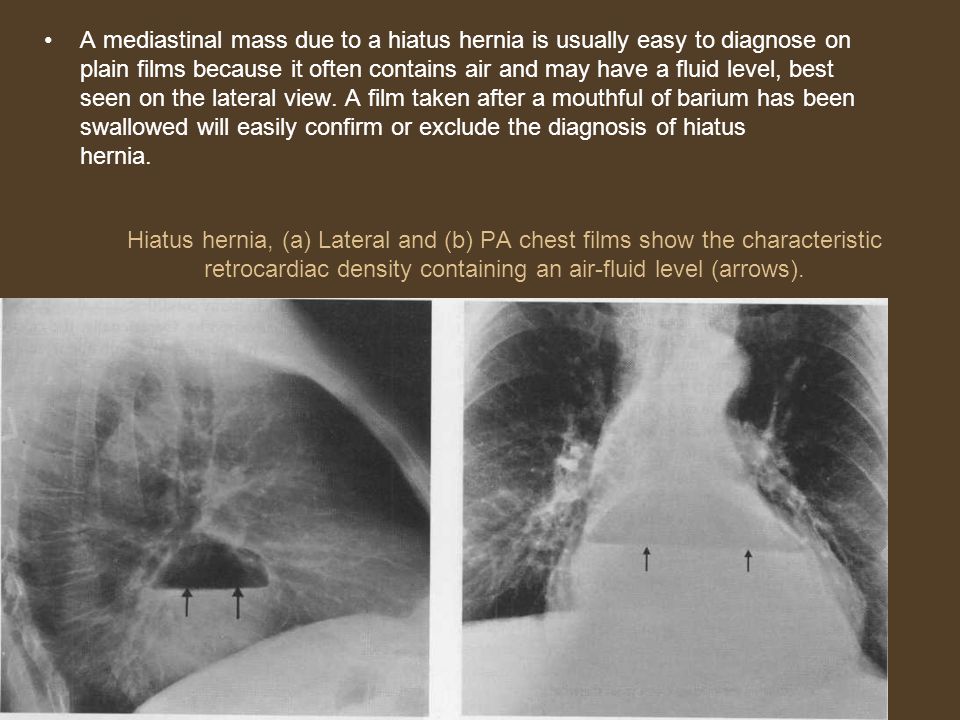The image appears to be an infographic from a medical textbook focused on diagnosing a mediastinal mass due to a hiatus hernia. The background is a medium to dark brown at the top, covering almost half the image, and extending down the right side by about a centimeter. The top text, in white Comic Sans font, reads: "A mediastinal mass due to a hiatus hernia is usually easy to diagnose on plain films because it often contains air and may have a fluid level best seen on the lateral view. A film taken after a mouthful of barium has been swallowed will easily confirm or exclude the diagnosis of hiatus hernia."

Beneath this, in tan text, it states: "hiatus hernia (a) lateral (b) PHS films show the characteristic retrocardiac density containing an air-fluid level (arrows)."

The infographic includes two black and white X-ray images on either side, divided by a vertically aligned rectangle about a centimeter thick. The X-ray on the right prominently features what appears to be a bone in the foreground, possibly surrounded by lung tissue with visible rib lines arcing diagonally. There's nebulous material at the base of the bone and a white object across the bottom, likely part of the bone structure. The background shows a black and gray gradient near the center bone. 

On the left X-ray, an arc of semi-opaque white color extends from the middle right edge up to the upper left and then diagonally down to the bottom right corner, suggesting layers of translucent, cloth-like material. Small black arrows point upwards in the center of each X-ray, indicating areas of interest related to the diagnosis of the hiatus hernia. The detailed text and images collectively demonstrate the typical radiographic features used to identify a hiatus hernia.